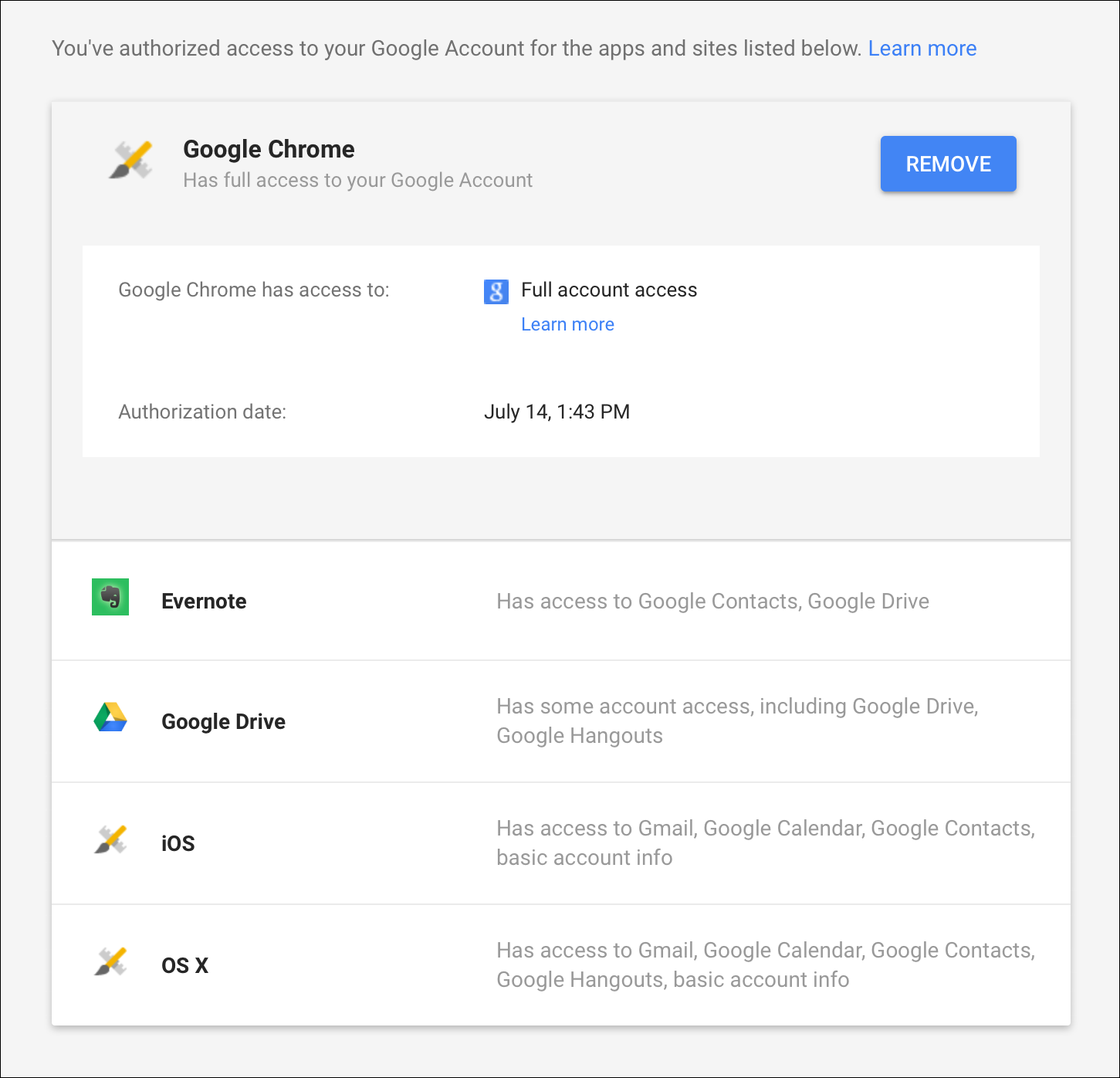A screenshot displaying authorized access to various applications on a Google account. The image shows a grey background highlighting four distinct sections of authorization details. 

In the first section, a blue rectangle labeled "Remove" indicates that Google Chrome has full access to the Google account, with the authorization date marked as July 14th, 1:40 PM. Moving to the second section, a green square and yellow fences depict that Evernote has access to Google Contacts and Google Drive. 

The third section exhibits a mix of green, yellow, and red elements, indicating access to Google Drive and Google Hangouts. A brush icon is also visible here. Finally, the last section details iOS's access to Gmail, Google Calendar, Google Contacts, and Basic Account Info, alongside Office Access, which similarly has permissions for Gmail, Google Calendar, Google Contacts, Google Hangouts, and Basic Account Info. Each section clearly outlines the extent of the authorized data access permissions for the respective applications.